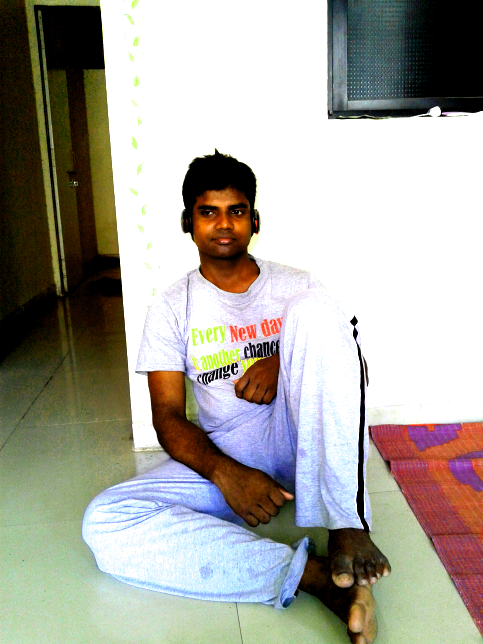The image depicts a young Indian man with dark skin and black hair, sitting on the ground and leaning against a white wall. He has on long, light blue pants with a stripe down the left leg and a light gray t-shirt with multicolored text that includes phrases like "every new day is another chance" alongside words such as "change" and "courage." He is barefoot, with the bottom of his feet appearing notably lighter than the rest of his skin. He is seated with his left knee elevated and his left foot resting atop his right foot, which lies flat on the ground. He has headphones on and is looking away from the camera with a neutral expression on his face. His left hand is folded across his chest while his right hand extends to the floor between his legs. Behind him, to his left, there is a hallway leading to a yellow door with a brown wooden border. To his right on the floor is a colorful rug featuring hues of red, orange, and purple, and above his right shoulder is a wall vent.